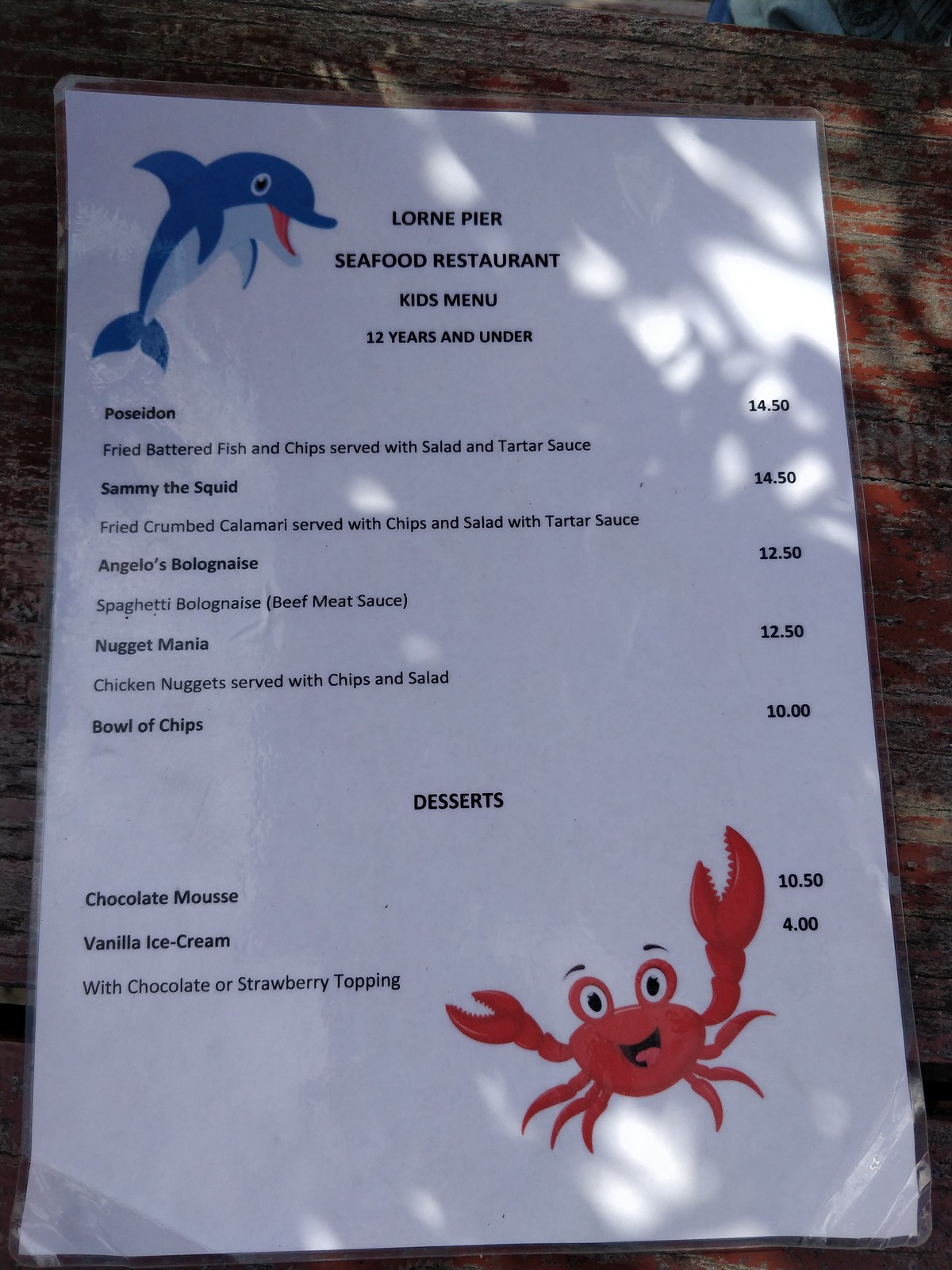In this photograph, a laminated kid's menu from Lorne Pier Seafood Restaurant is displayed neatly atop a weathered wooden picnic table, suggesting the shot was taken outdoors. The table's faded red paint, now mottled and worn, adds a rustic charm to the scene. The menu, designed for children aged 12 and under, features a playful layout with a white background adorned with two cartoon characters—a dolphin at the top left and a red crab at the bottom. The menu lists various kid-friendly food options, including a bowl of chips, chicken nuggets, spaghetti, calamari, and fish and chips, alongside a brief dessert section. The outdoor setting is hinted at by the shadows cast over the menu, indicating a natural light source with some sun filtering through.